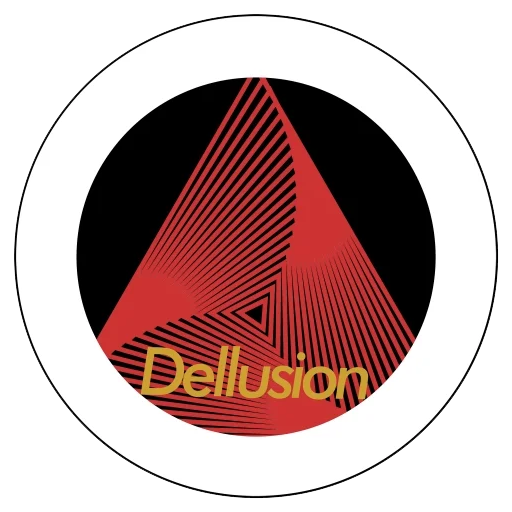The image features a striking graphic design, presenting a central red and black stylized triangle with a wavy, abstract pattern. This triangle, positioned in the middle, extends outward in three directions resembling outspread wings, and is integrated within a circular motif. Surrounding the triangle is a black background, encased within two concentric circles: an inner band of white and an outer ring of black. The design prominently displays the text "DELUSION" at the bottom center within the black background, spelled uniquely as D-E-L-L-U-S-I-O-N, with a capital 'D'. The bold yellow text contrasts sharply against the black, enhancing its visibility. Overall, the intricate composition suggests a potential logo for a company or product, combining elements of geometric abstraction and dynamic movement.